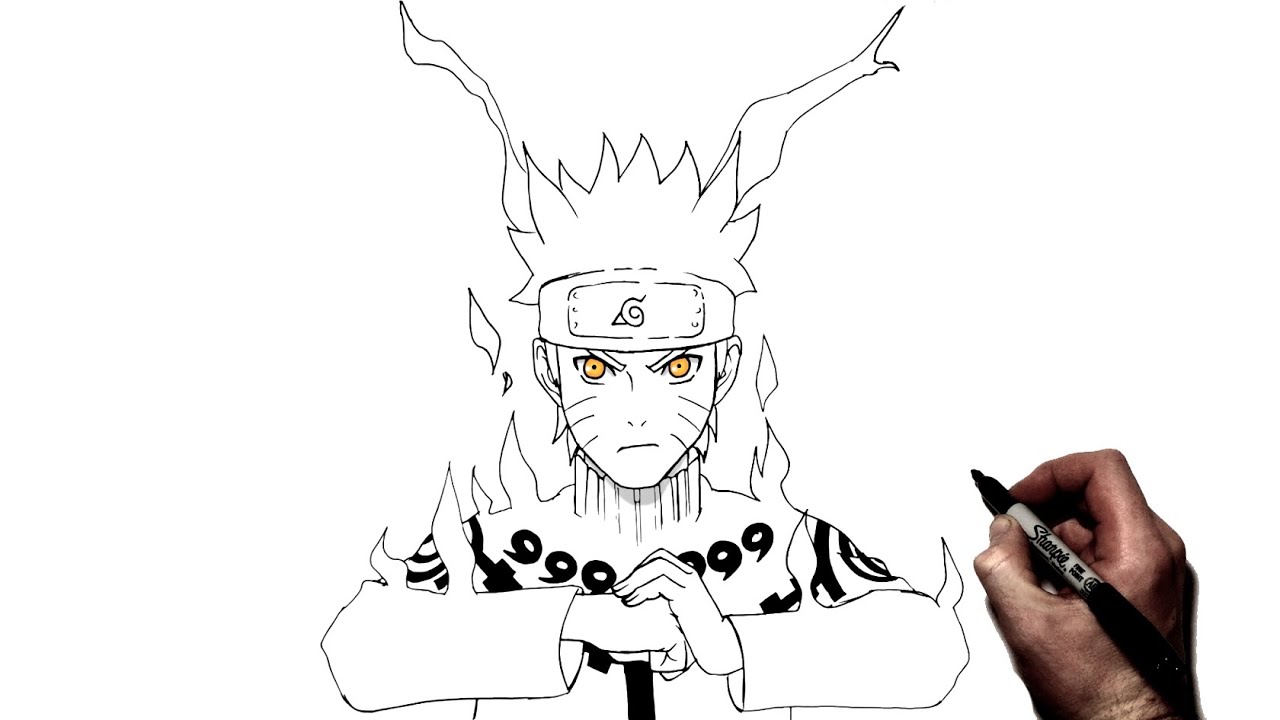In this image, we see a human hand, visible from the wrist up, holding a black Sharpie with a grey body and "SHARPIE" written on it in black. The hand is actively engaged in sketching an anime cartoon character on a piece of paper. The anime character depicted is a young man with distinctive features: three scars on both sides of his face, gold cat-like eyes, and whiskers. He wears a detailed headband bearing a spiral shape with an outer triangle and a flame-like helmet. Emerging from the helmet are horn-like protrusions. His shirt displays the number 9 repeated six times on the collar and various symbols adorning the shoulders. Fire-like brush strokes rise from the base of his cape, contributing to the dynamic and fierce expression on his face. His hands are drawn in a traditional martial arts stance, with one fist clasped into the palm of the other, as though he is preparing for a fight. The intricate details of the character, especially the unique elements like the upside-down sixes, antlers, and whiskers, emphasize the artist's skill and the character's intense persona.